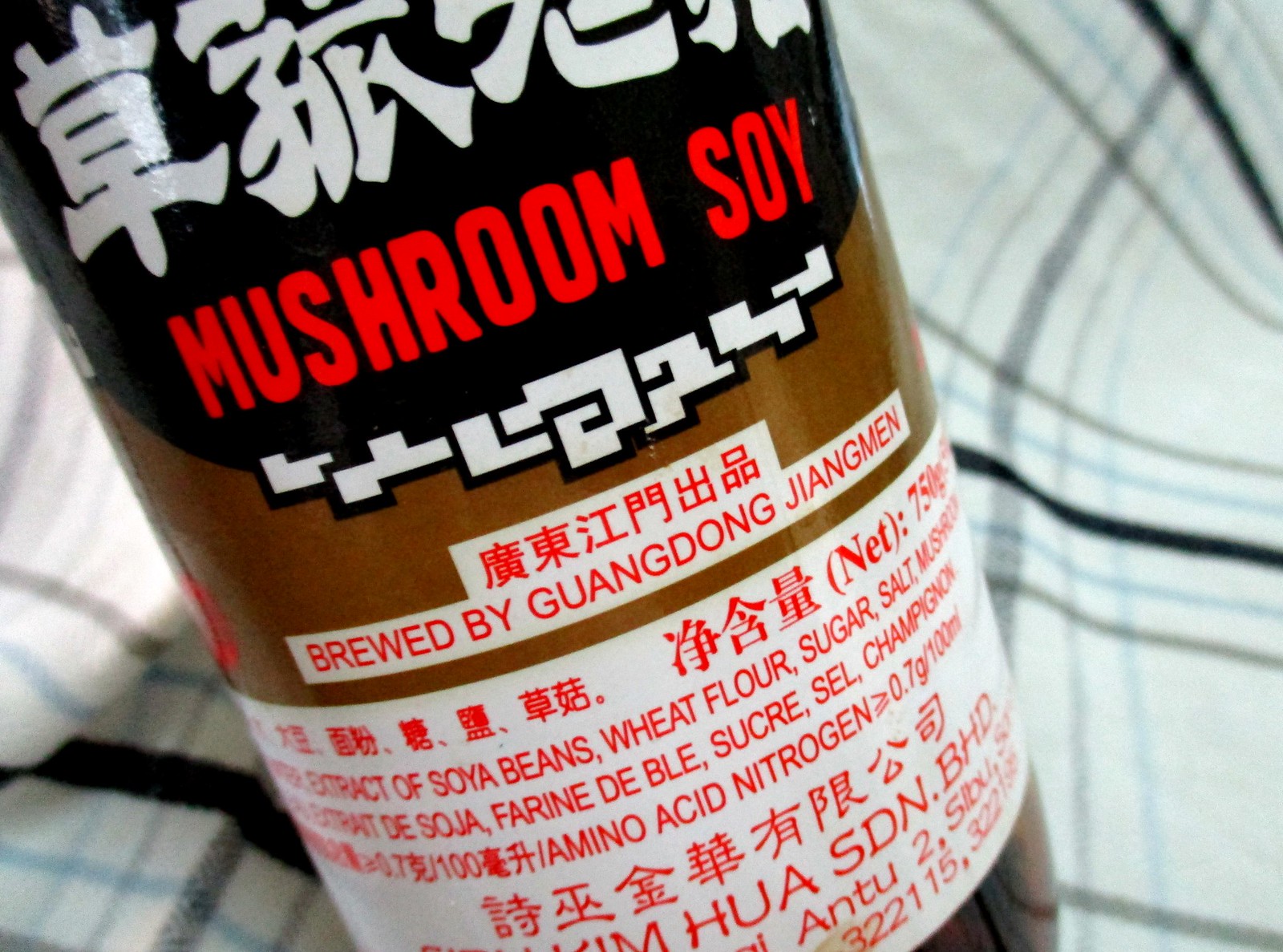The image shows a close-up of a mushroom soy sauce bottle against a plaid fabric background. The bottle features a black label at the very top adorned with Chinese characters in white, and beneath that, the words "mushroom soy" are prominently printed in red. Below the main label, there is a series of smaller inscriptions, including Tetris-like symbols and intricate scrolls, alongside a white border with more red Chinese characters. The text underneath reads "brewed by Guangdong Young Men" (names vary but suggest a similar interpretation). Further down, an additional large white label includes the ingredients list: extract of soya beans, wheat flour, sugar, salt, mushroom, and details about the amino acid nitrogen content. The plaid fabric in the background hints that someone might be holding the bottle, adding an informal touch to the detailed presentation.